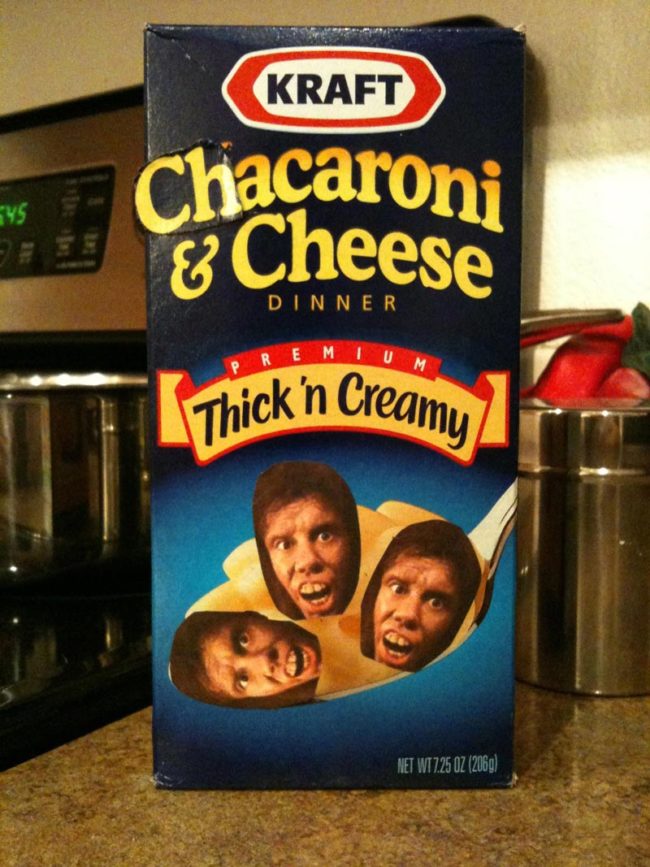In this whimsical kitchen scene, a box of Kraft Macaroni & Cheese sits prominently on the countertop, positioned near a stove with a pot to the right. The box has been humorously altered: the original "Macaroni" has been changed to "Chacaroni" by pasting "CH" over the "M" in a matching font style. Adding to the satirical flair, three photos of a person with a peculiar, caveman-like face, featuring artificial teeth and a strange haircut, are pasted over the spoonful of macaroni on the box. These images are arranged at the 9 o'clock, 12 o'clock, and 3 o'clock positions, turning the everyday food item into a comical and whimsical meme. The label at the bottom still reads "Premium Thick and Creamy," adding to the blend of absurdity and reality.